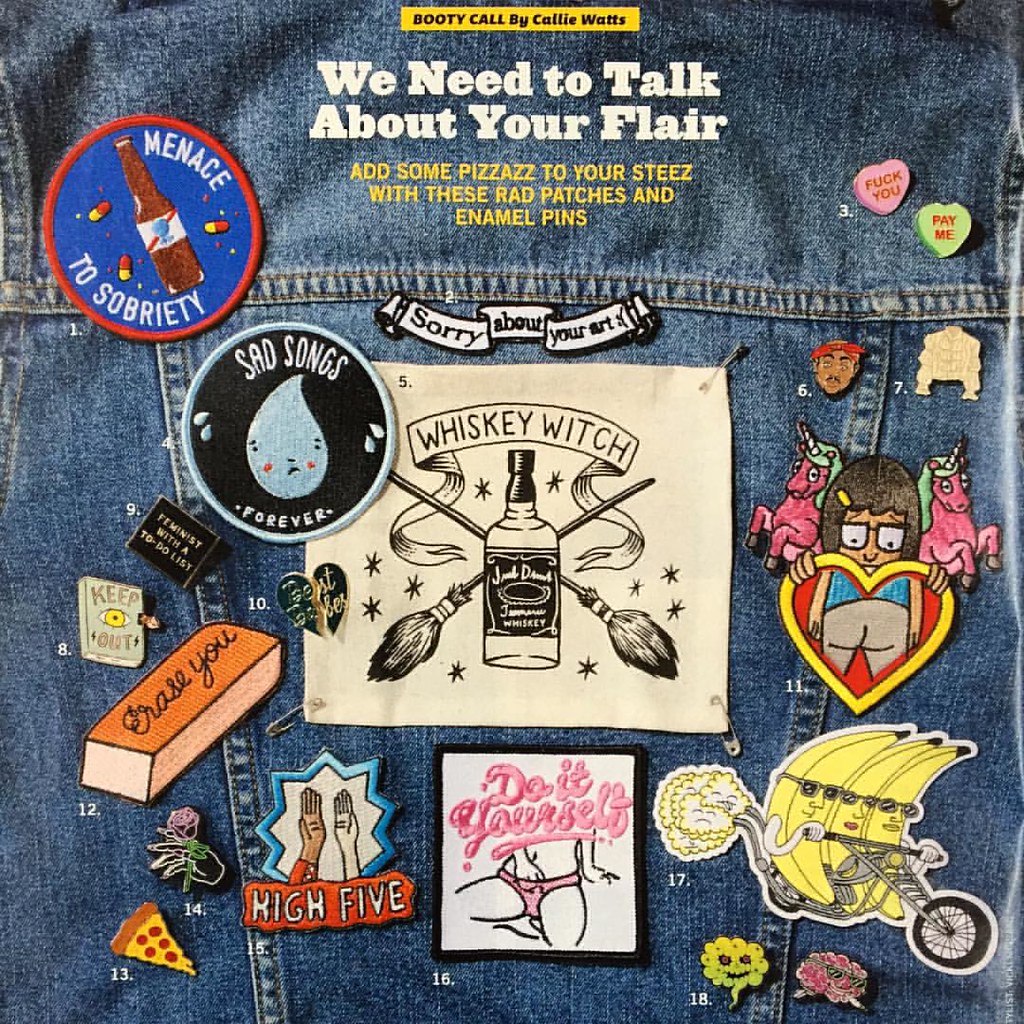The image is a highly detailed, close-up photograph of the back of a denim jacket adorned with 18 vibrant, embroidered patches and enamel pins, each with unique and often cheeky messages or designs. The upper center of the image features a yellow box with the title "Booty Call by Callie Watts," followed by white text stating, "We need to talk about your flair," and yellow text below reading, "Add some pizzazz to your steez with these rad patches and enamel pins."

Prominent patches include a central square patch that declares "Whiskey Witch," featuring a bottle of Jack Daniels illustrated in black pen over crossed broomsticks. Nearby, a circular patch reads "Menace to sobriety" with imagery of a beer bottle and pills. Another notable patch shows candy hearts inscribed with "Fuck you" and "Pay me." There is also a feminist-themed patch with a to-do list and a humorous "Do it yourself" patch depicting a woman putting her hand down her panties.

Flanking these patches are a variety of other designs, including a patch emblazoned with "Sad songs forever" accompanied by a sad water drop, a "Feminist" patch, a "Keep out" tag, a "Erase you" patch, a rose, a slice of pizza, a high-five icon, and a trio of cartoon bananas riding a motorcycle. Additional whimsical patches feature flowers, Tupac caricatures, and unicorns paired with a girl's bottom. The jacket, possibly an advertisement or a well-curated photograph, serves as a playful canvas to showcase these eclectic and often irreverent designs, inviting viewers to personalize their style with these bold accessories.